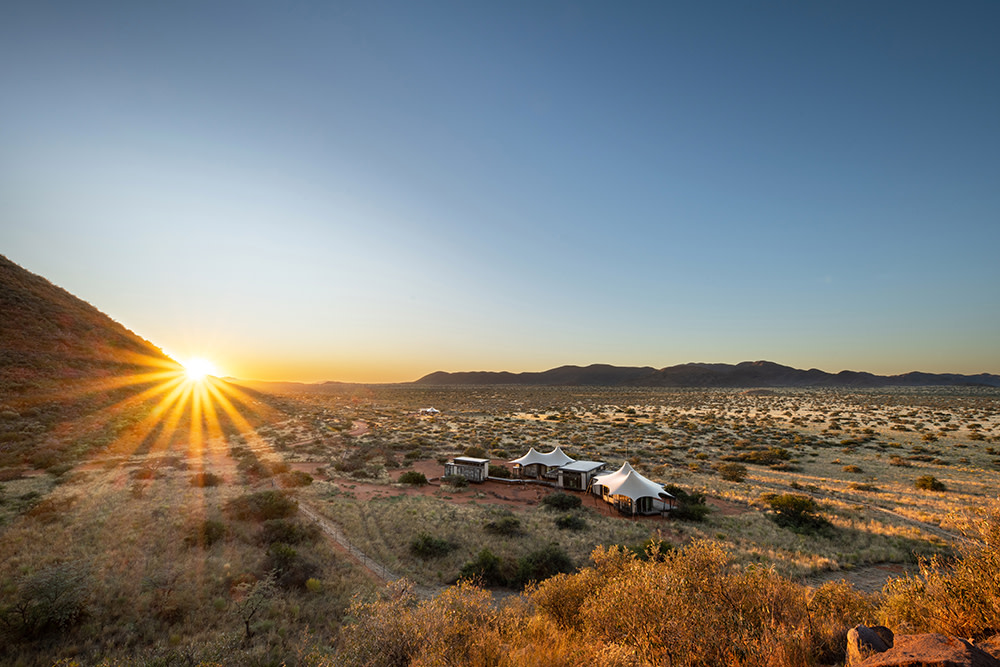This photograph captures a serene desert landscape during the golden hour with the sun setting behind a gentle, steep hill on the left side of the image, casting an array of beaming sun rays across the scene. The foreground features a dry, sandy terrain dotted with small bushes and shrubbery. In the center of the image, there are four distinct structures with white roofs, two of which are pointed while the others are flat. These buildings appear to be either homes or tents. Beyond these structures, a faint image of a white pickup truck can be seen. In the distance, the horizon is defined by low, dark-colored hills on the right, creating a stark contrast with the lighter tones of the foreground, while the sky transitions from a grayish hue to golden near the setting sun.